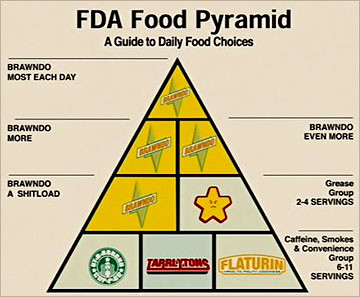This image features a satirical rendition of the FDA Food Pyramid, labeled "FDA Food Pyramid: A Guide to Daily Food Choices" in black text at the top. The pyramid is divided into several sections, each accompanied by humorous and exaggerated food recommendations. 

At the very peak of the pyramid, the text reads "Brondo, most each day." Directly below this, the next section repeats the word "Brondo" with increasing quantity annotations: "Brondo more" and "Brondo even more." 

The third tier humorously exaggerates further with the phrase "Brondo a shitload," and also includes a category labeled "grease group, two to four servings." Closer to the foundation of the pyramid, a section labeled "caffeine, smokes, and convenience group" prescribes an excessive "six to 11 servings."

The base of the pyramid humorously displays parodied logos of well-known brands, including a spoof of the Starbucks logo among others, adding a layer of satirical commentary on modern dietary choices. This image clearly serves as a humorous critique of dietary guidelines and contemporary eating habits.